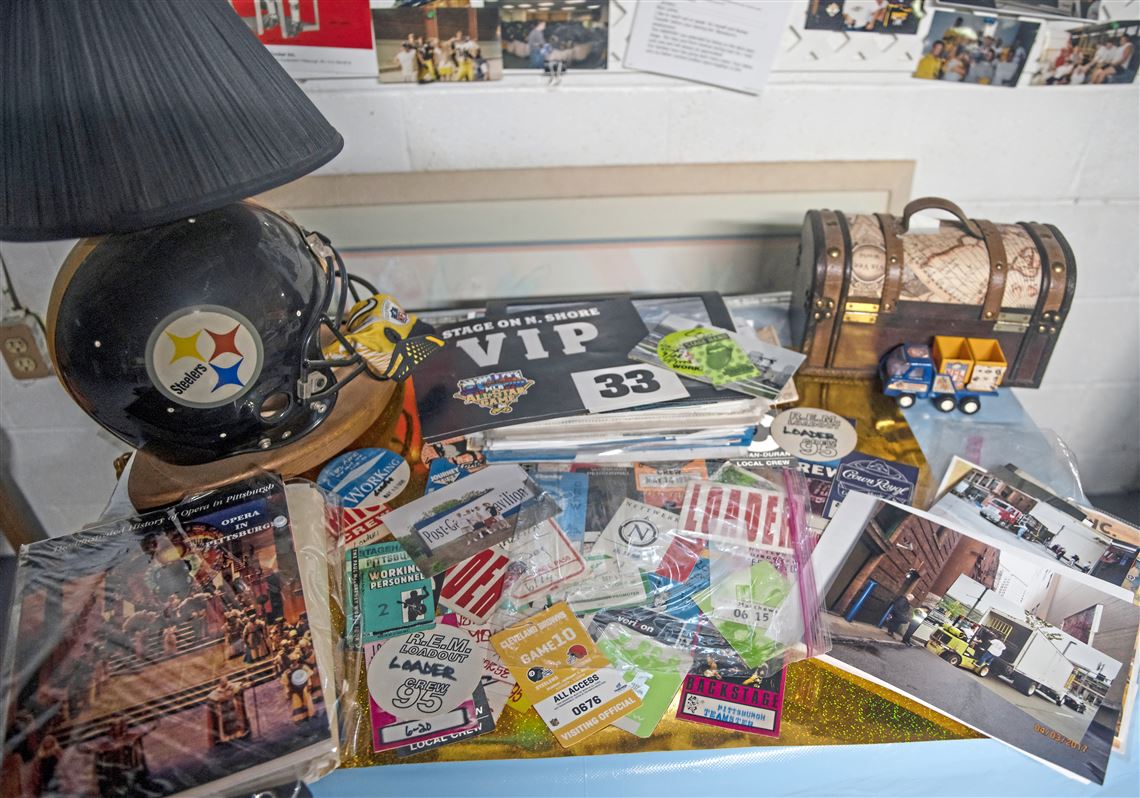The image depicts a desk brimming with memorabilia that reflects the interests and passions of a Pittsburgh Steelers fan. Centered on the desk is a distinctive black lamp fashioned from a Steelers helmet, adorned with a black shade showcasing the team’s emblem. A collection of items is scattered across the surface, including a vivid snapshot of Pittsburgh's cultural scene captured in an opera magazine or brochure.

A small chest-like decoration is positioned on the right side, beside a toy truck loaded with two boxes on its flatbed, echoing scenes of labor depicted in some of the photographs on display. One notable picture shows a forklift lifting cargo into a semi-truck, dated 4-3-2017, while another features four men together. There are numerous tickets and stickers strewn around, including a blue VIP ticket labeled "Stage Onshore VIP Number 33" for the All-Star Game, a ticket for a Cleveland Browns game numbered 10, and an "All Access Pass". Memorabilia fans might notice a sticker that reads "REM, lead out leader, crew 95", adding to the eclectic mix of collectibles. These various items, including the thematic stickers and football-related trinkets, evoke a sense of cherished memories and heartfelt fandom.